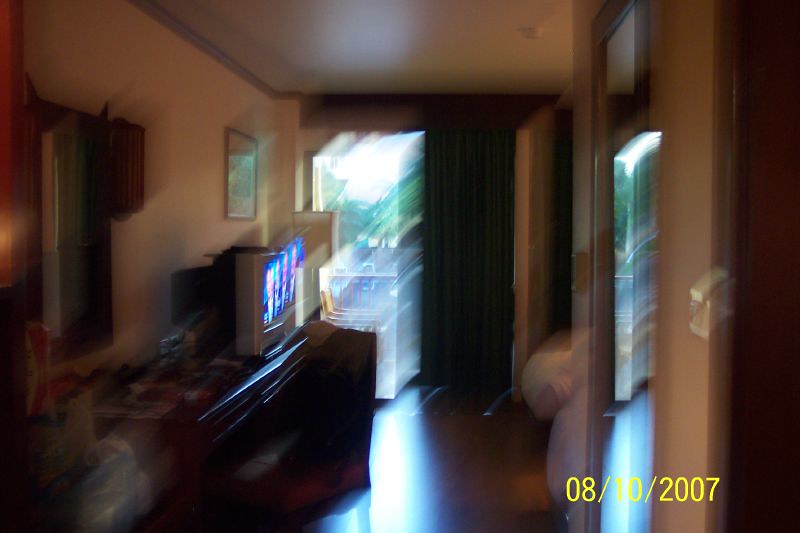The blurry, retro-styled photograph depicts a living room or possibly a bedroom from the perspective of the doorway. On the left side, against a brown wooden desk or TV stand, sits an old-fashioned, boxy television displaying a person with a blue background, likely a newscaster. The TV is notable for its bright screen and the date 8-10-2017 displayed in yellow in the bottom right corner, resembling the style of an old camcorder.

Near the TV stand, there are items that suggest it might also function as a dressing table, featuring drawers and a padded chair. Above the stand, there's a small mirror with a wooden frame. On the right side of the image, a tall, stand-alone lamp with a long pole and a lampshade is visible. Further to the right, part of a wooden cupboard or closet door can be seen.

The far right shows what might be the bottom of two single beds or a couch. In the background, there is a sliding door or large window leading out to a balcony or deck. Daylight streams through, illuminating green trees and a small table outside, indicating it is daytime. The interior and exterior elements, along with the various household items, create a sense of a lived-in, personal space caught in a moment of time.